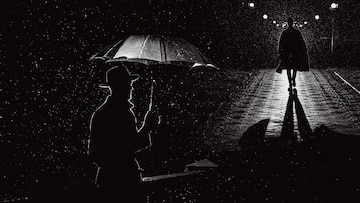This small rectangular black and white photo captures a dark, rainy, nighttime scene defined by its stark contrasts and silhouette. Central to the composition, a man in a hat and trench coat stands holding an umbrella, his form illuminated subtly around the edges by the scant streetlights, giving his figure an almost ethereal glow. A glossy walkway stretches out in front of him, where another man, also in a long trench coat and hat, walks away into the darkness, casting a pronounced shadow behind him. Lights strung delicately on both sides of the walkway add a fragmented illumination, contributing to a tense, mysterious atmosphere. The overall scene feels gloomy and eerie, evocatively capturing a moment thick with suspense and the unknown, framed by dark shapes and the shimmering wet street.